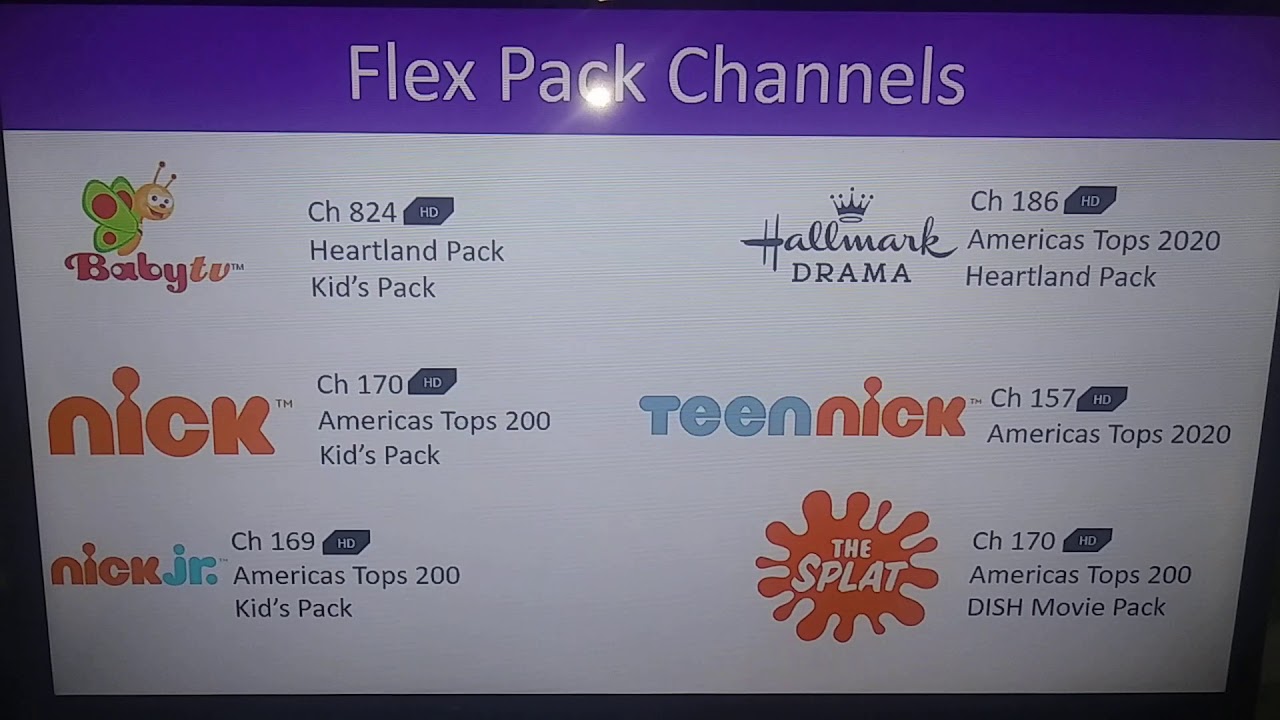The image is a photograph of a screen or placard displaying channel listings for FlexPak. The header at the top of the screen is highlighted in blue, while the remainder of the screen is white. A camera flash is visible, indicating this was a photo taken with a flash on.

The detailed channel listings displayed are as follows:
- **Baby TV** - Channel 824, available in the Heartland Pack and Kids Pack.
- **Nick** - Channel 170, included in America's Tops 200 and Kids Pack.
- **Nick Jr.** - Channel 169, part of America's Tops 200 and Kids Pack.
- **Hallmark Drama** - Channel 186, found in America's Tops 2020 and Heartland Pack.
- **Teen Nick** - Channel 157, featured in America's Tops 2020.
- **The Splat** - Channel 179, present in America's Tops 2020 and Heartland Pack.
- **The Splat** (possibly a duplicate or another listing error) - Channel 170, mentioned under America's Tops 200 and Dish Movie Pack.

The list suggests an emphasis on children's programming and family entertainment, available across various channel packs and listings for the FlexPak service.